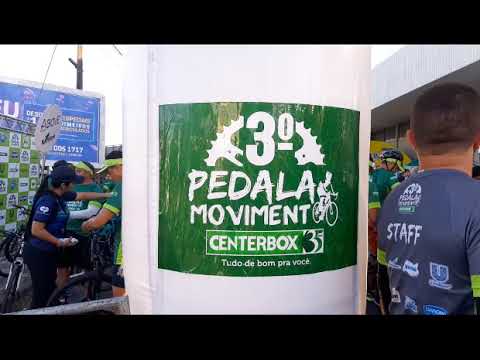The image captures an outdoor setting under a grey sky with a central white column bearing a green sign. The sign prominently features white text that reads "Free Zero" at the top, followed by "PEDALA" in bold, and then "MOVIMENT." There is also a white silhouette of a person riding a bike. Just below this, the sign says "Centre Box" in white text. The left section of the image shows several people, some in green bike shirts and lime green visors, appearing to be at a stand handing items out. Among them, a woman with long black hair is seen wearing a blue top and black pants. The right side of the image includes a man in a dark grey T-shirt labeled "Staff" in white text, facing away from the camera, with additional bicyclists surrounding him.